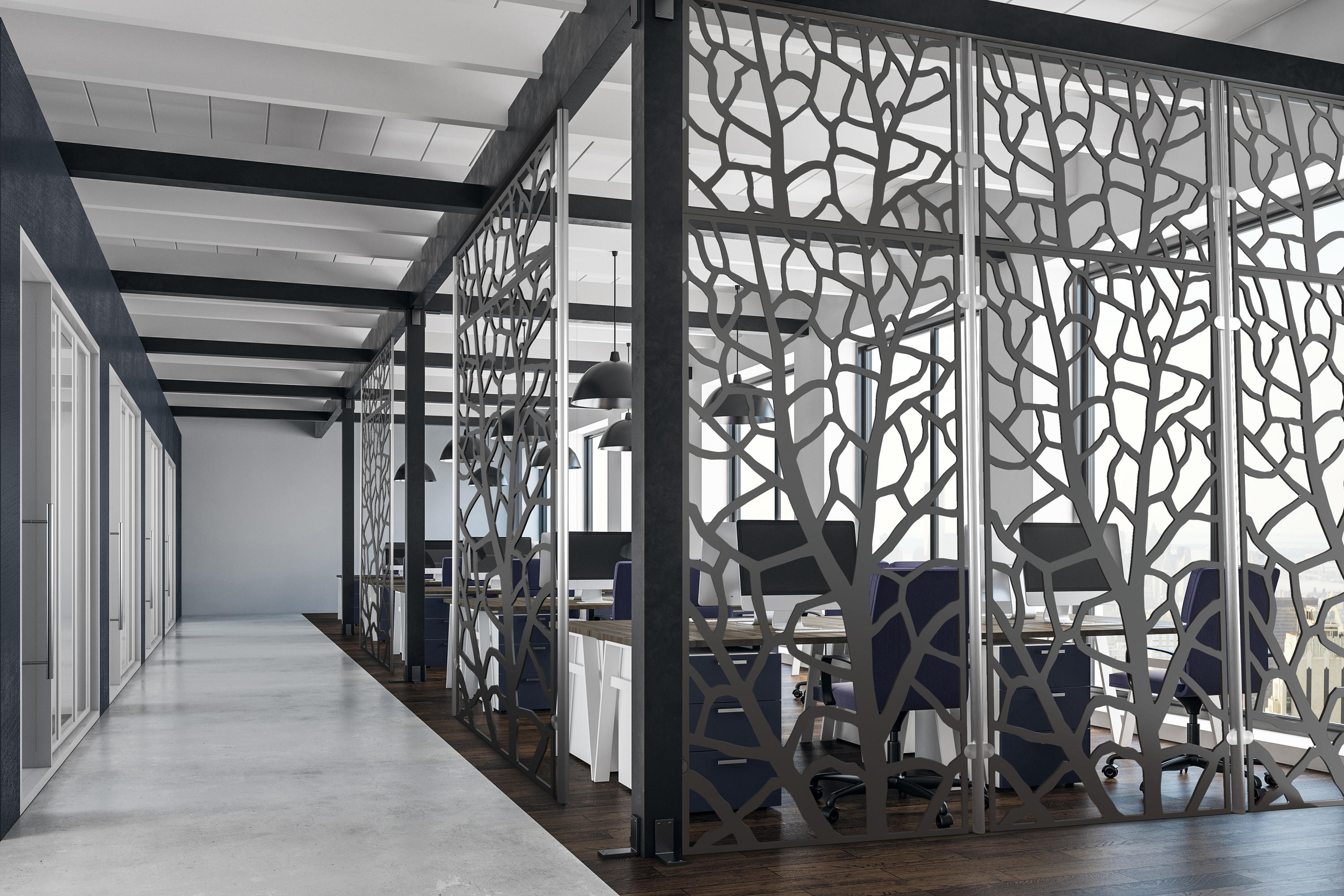This image depicts a clean, modern office space with distinct design elements. The room features both a marble-like light gray stone flooring on the left side, and dark hardwood flooring on the right side that stretches throughout most of the area. The left side is characterized by a narrow strip, about three feet wide, running adjacent to a row of large windows that allow ample sunlight to illuminate the interior. 

On the right side, approximately ten feet wide, are several desks each equipped with computer monitors and complemented by gray or blue file cabinets and blue desk chairs. The desks are arranged cubicle-style and are separated by unique metal dividers designed to resemble tree branches, adding a touch of natural elegance to the space. 

The walls of the office are predominantly white, although the back of the hallway extends towards a gray wall. The ambiance is both humble and modern, creating a well-lit, inviting workspace.